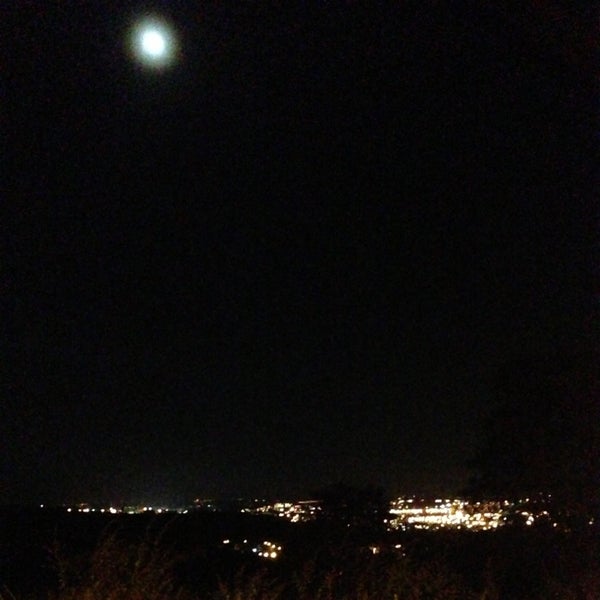This nighttime photograph captures a panoramic view of a city from a great distance, enveloped by a dark night sky. Dominated by a deep black color, the sky showcases a hazy, slightly blue-tinged moon shining from the upper left corner. Below the moon, the vast expanse of the sky gradually transitions to a bustling cityscape in the bottom horizontal quarter of the image. The city lights, scattered across the scene, are most concentrated on the right and gradually diminish toward the left, where they become sparse. In the foreground, some trees and shrubs slightly obstruct the view. The brightly lit buildings, primarily low and horizontal, appear to be around three to four stories high, with their illumination providing the main highlights against the otherwise starless sky.